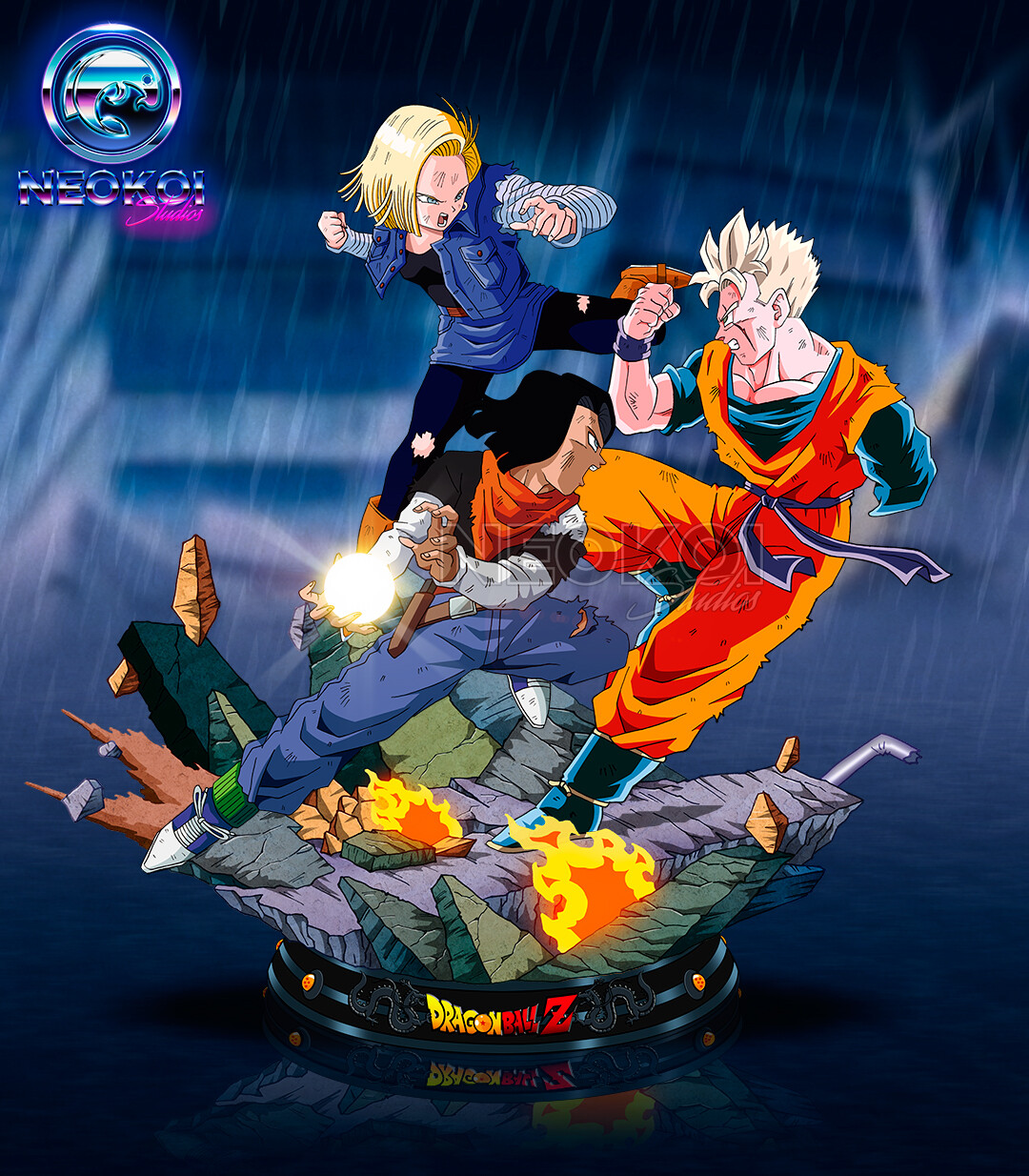In this detailed graphic, set against a rainy, slightly out-of-focus blue background with gray and light-blue designs resembling the side of a building, three figures from the Japanese animated program Dragon Ball Z are depicted mid-battle. At the top left of the image, a metallic-looking badge bears the label "NEO KOI" in shiny modern lettering of blue, silver, and purple. Below this, the iconic "Dragon Ball Z" logo is displayed prominently in yellow and red letters at the bottom center. 

In the graphic's foreground, we see an intense combat scenario involving three characters. On the right, a white male with spiky bleached blonde hair donning an orange jumpsuit—missing one arm, evident by the empty blue sleeve—faces off against two opponents on the left. The first is a blonde-haired Caucasian girl in a gray and blue outfit that includes a blue skirt and torn black leggings, who is launching an attack while holding a glowing orb in her right hand. Above her, another figure—described variously but seems to overlap with the description of a man in blue jeans and an orange handkerchief—jumps in, delivering a kick. They all stand on a rocky surface with swirling orange and yellow flames underneath them, framing the chaotic energy of the scene.